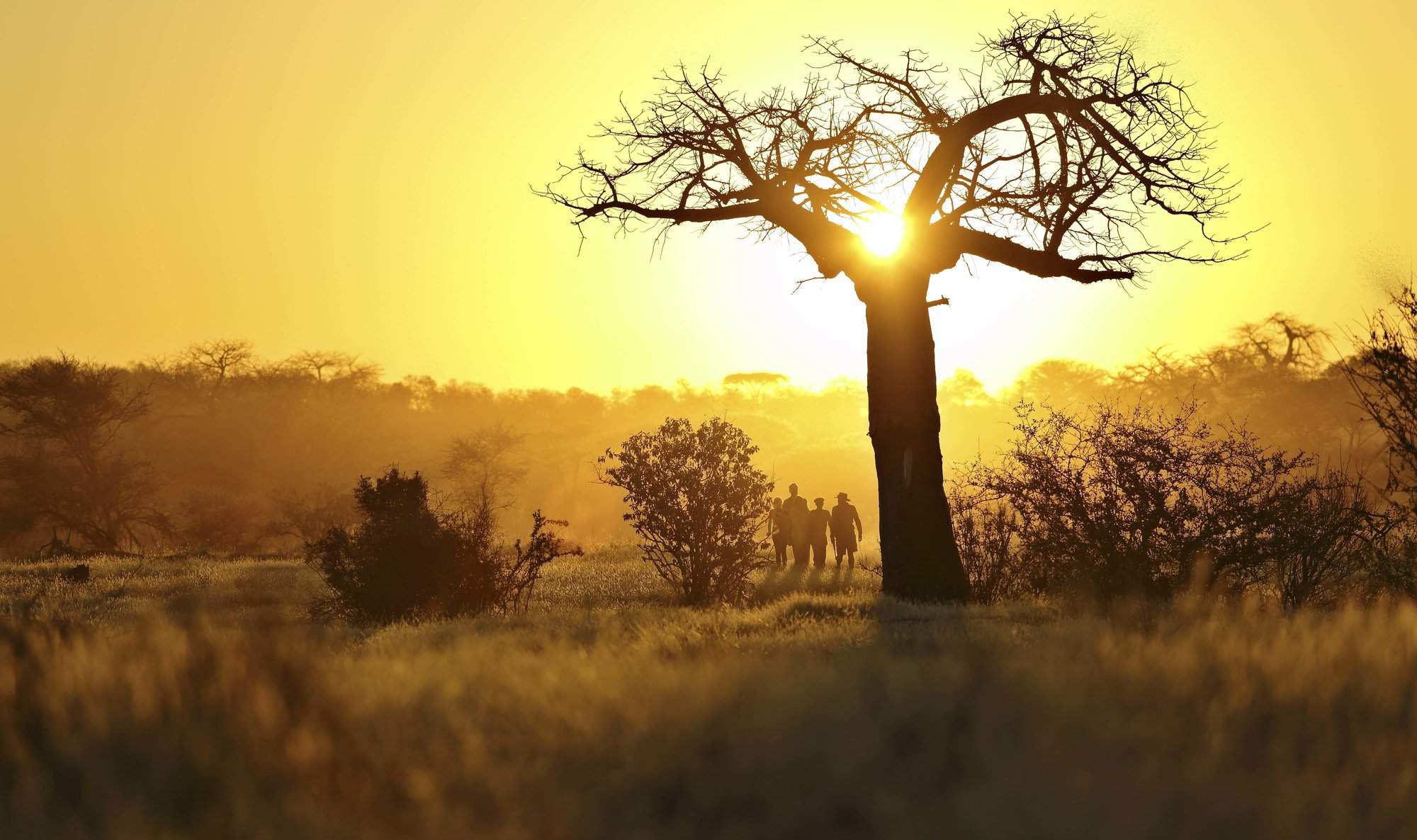The image depicts a vast, open landscape bathed in the warm hues of either sunrise or sunset, casting a predominant yellow and orange glow across the scene. At the center stands a large, prominent tree with a bare trunk that branches out at the top in a tangled web. The tree is bathed in silhouette, starkly black against the bright, glowing sky. Around the base of the tree, the ground is sprinkled with various bushes and grasses, both thorny and non-thorny, adding texture to the landscape. To the left of the tree, four silhouetted figures stand close together, their nondescript forms suggesting they are either looking towards the vibrant sunset or the majestic tree. Further into the background, the silhouettes of a distant forest are faintly visible, adding depth to the scene and emphasizing the rich, safari-like environment. The overall color palette is dominated by black, yellow, and hints of orange, giving the image a striking and serene ambiance.